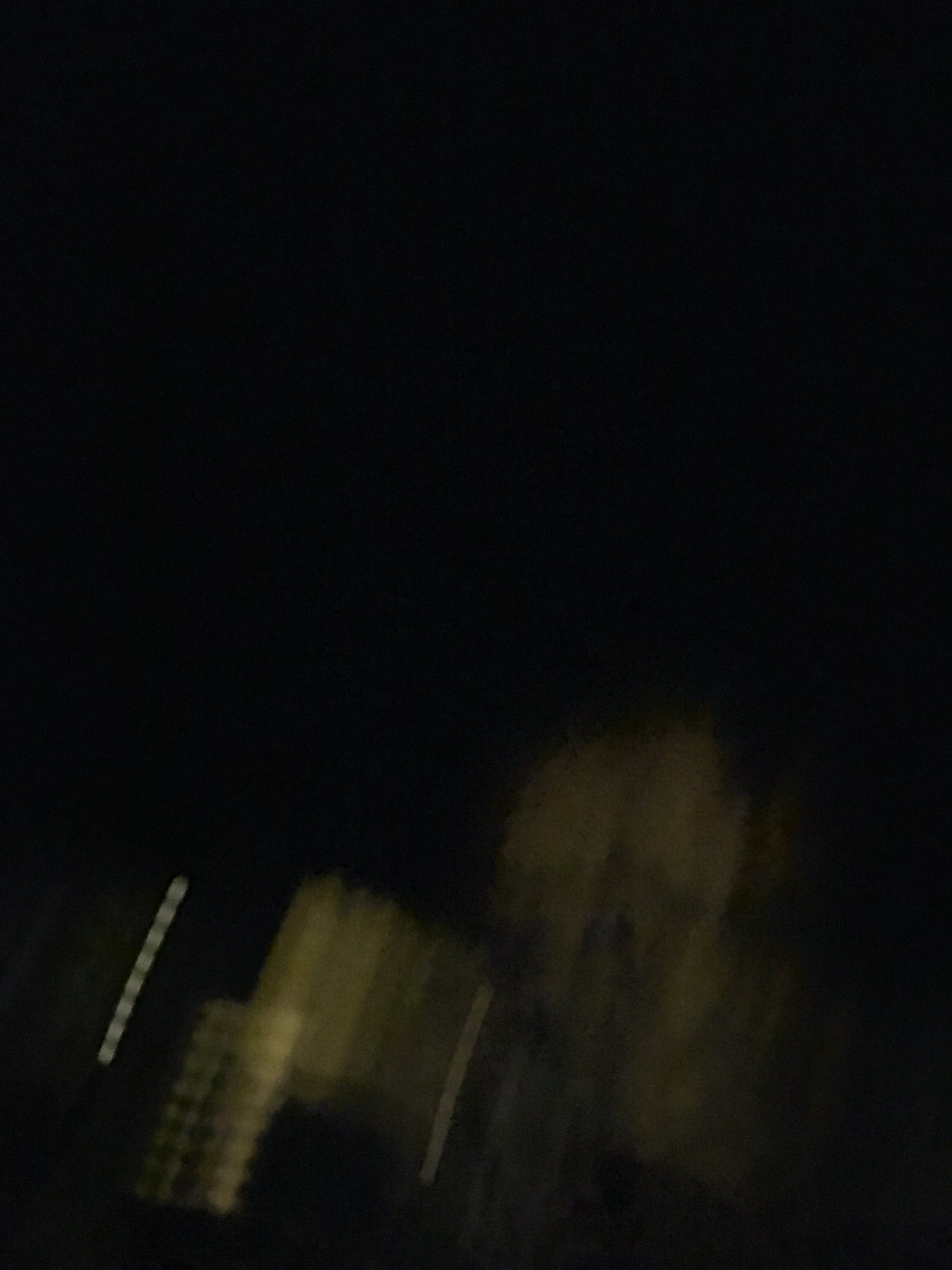This photograph captures a very blurry scene taken outdoors at night. The background is completely black, indicating the depth of the night sky. The indistinct object in the foreground, whose details are hard to discern due to the blurriness and low light, appears to be of a light cream color with areas of dark gray or black. Behind this object, multiple lights shine through the darkness, adding some definition to the scene. A vertical line of bright white lights stands out against the black background, while scattered panels of lights emit a warmer, goldish-white glow, adding a hint of warmth to the otherwise dark environment. The interplay of light and dark creates an elusive, almost abstract visual experience.